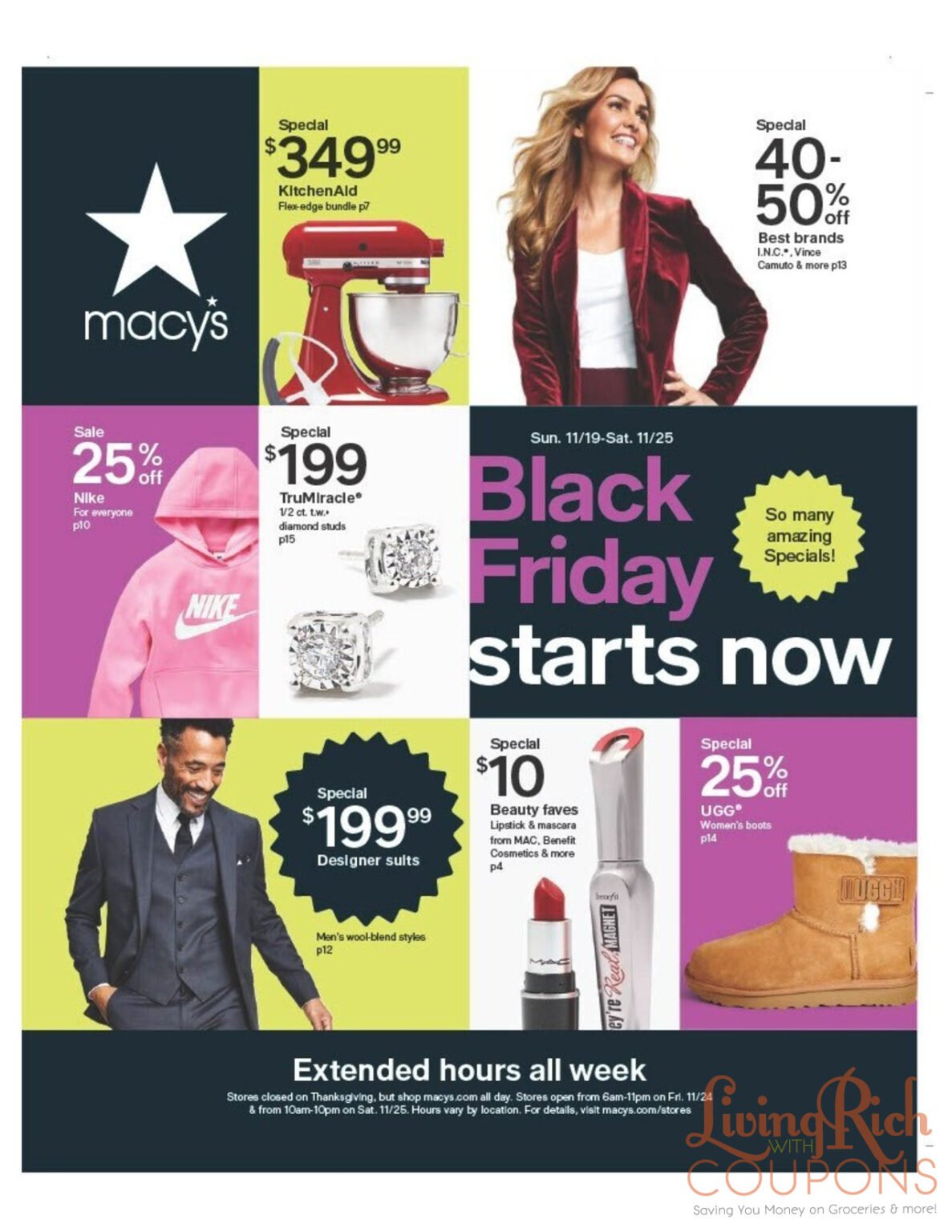This image is an advertisement for Macy's showcasing various sales and promotions. The layout is divided into colorful blocks, each highlighting a different deal. In the top left, the Macy's logo, featuring its iconic star, is displayed in white against a navy background. 

In the bottom right corner, there's a watermark from "Living Rich with Coupons," which emphasizes saving money on groceries and more, and features an orange and gray color scheme. 

Several promotions are detailed within the ad:
- On a green background, there's a special offer of $349.99 for a red KitchenAid mixer.
- Beside this, an image of a woman with blonde hair, wearing a white top and a red velvet jacket, advertises 40-50% off best brands.
- A purple block highlights a sale on a pink Nike hoodie with a white Nike logo, featuring a 25% discount.
- Another block showcases diamond-style earrings for $199, branded as "True Miracle."
- Below, a man in a black suit is featured with a special price of $199.99 for designer suits.
- Additional deals include $10 beauty favorites from MAC, Benefit Cosmetics, and more, as well as 25% off UGG women's boots.
 
The ad mentions Black Friday specials running from 11/19 to 11/25, with extended hours all week long.